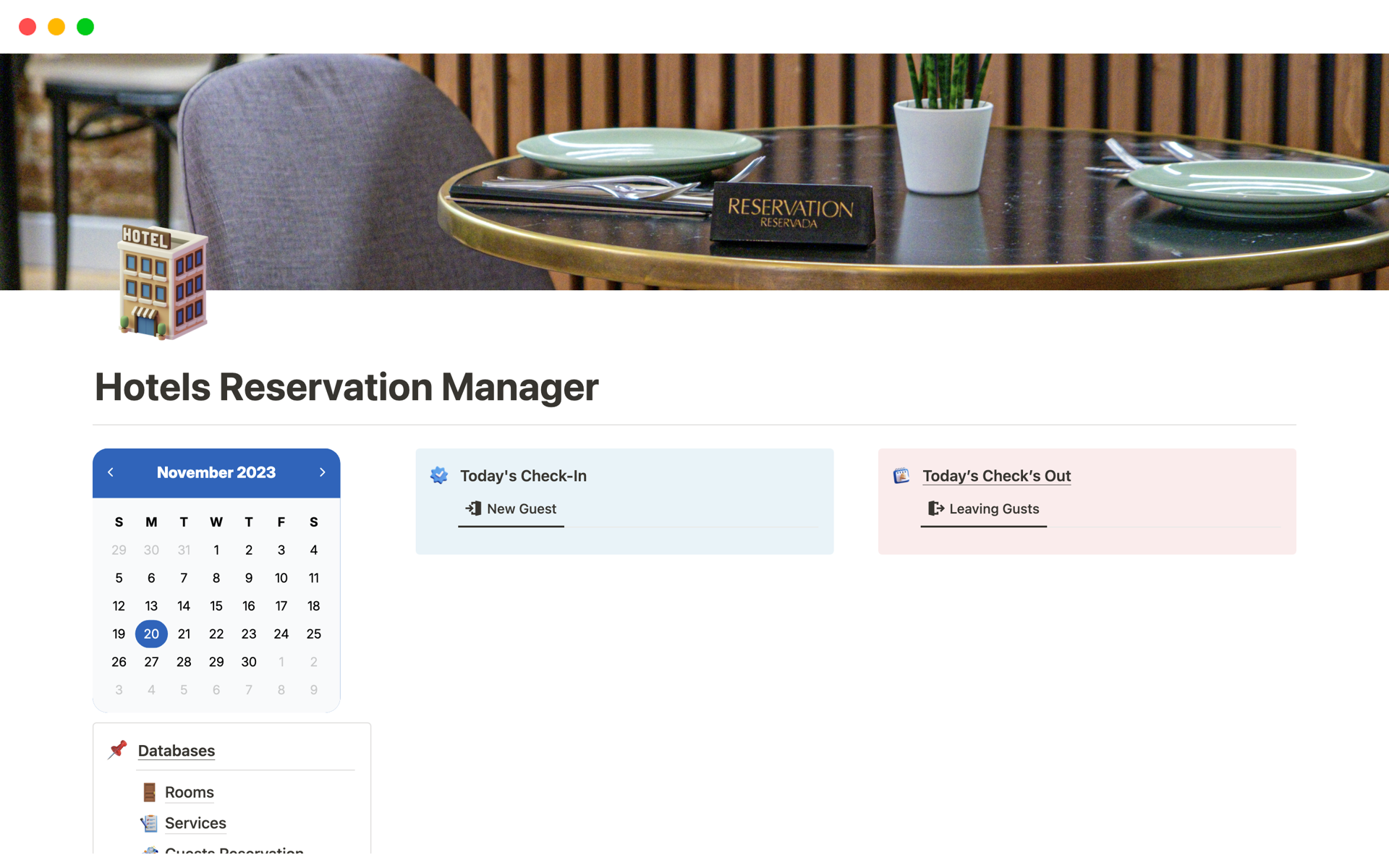The image is a horizontally oriented rectangular photo focusing on a glass table with a gold-trimmed edge, slightly cut off on the right-hand side. At the center of the table sits a green plant in a white pot, which is cut off at the top. Positioned to the right of the center of the photograph, the plant is surrounded by an elegant setting.

Two mint green plates are arranged on the table: one is placed at the center of the right edge, and the other is a little to the left of the midway point of the image. Each plate is accompanied by silverware neatly placed beside them.

In addition to the table setting, a dark-colored rectangular sign is prominently displayed on the table. Written across the center of the sign in gold font is the word "Reservation," with additional text beneath that is not fully visible. To the left of the chair at the table's edge is a small hotel icon. Below the icon, the text reads "Hotels Reservation Manager" in black font.

Adjacent to this is a vertical calendar for November 2023, featuring blue headers with navigation arrows on either side. The days of the week are marked in bold black font, and each day is represented by an initial, like "S" for Sunday and "M" for Monday. The 20th day is highlighted with a blue circle. A red push pin marks a section labeled "databases," with "rooms" and "services" noted alongside their respective emojis.

To the right of the calendar are two horizontal rectangular boxes. The first box, in baby blue, lists "Today's check-in" with "new guest" written underneath. The second box, in baby pink, displays "check-out" with "leaving guest" noted below.